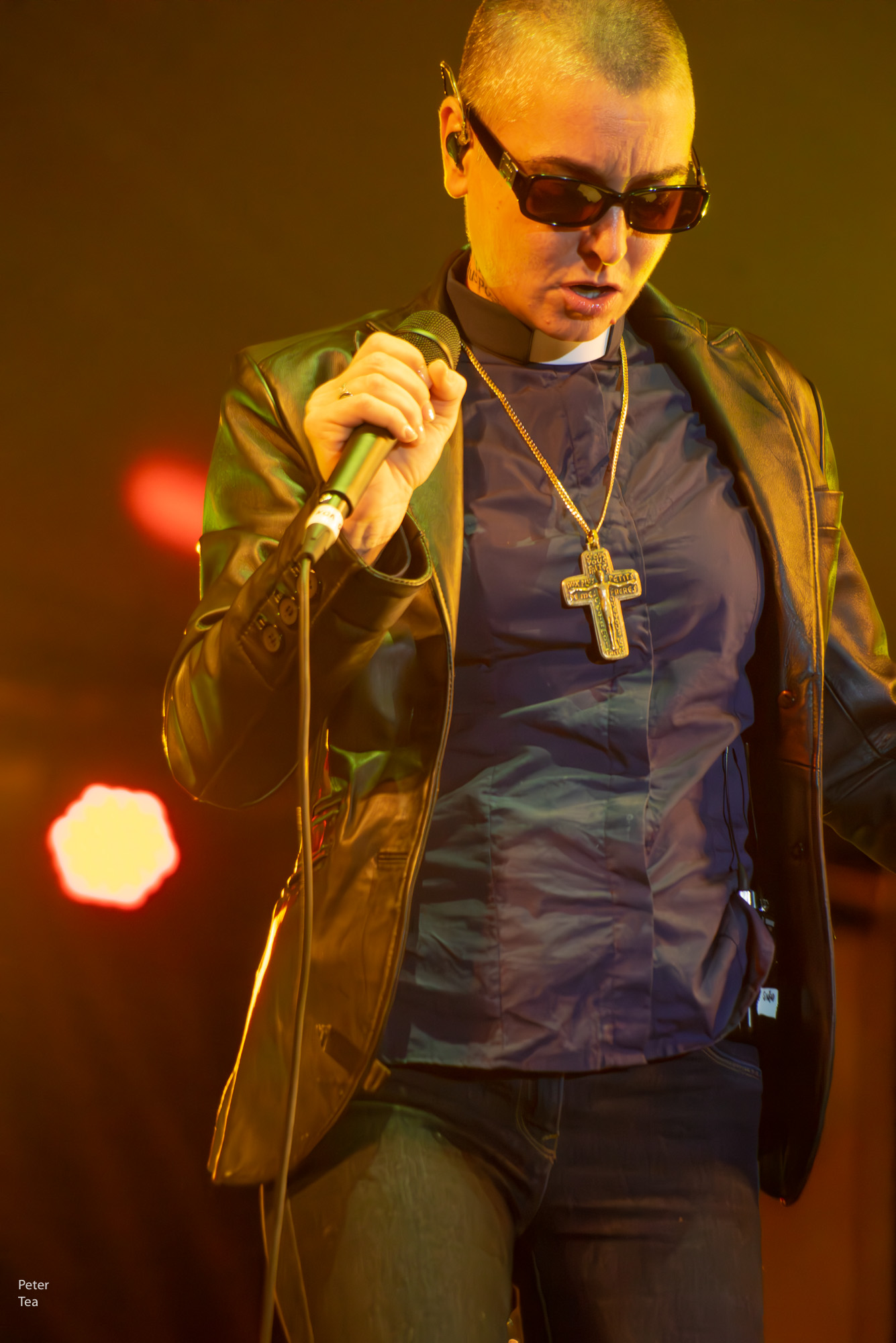The photograph captures a poignant moment of a woman, identified by some as Sinead O'Connor, on stage during a performance. She's framed from her upper thighs to the top of her head against a black background, with spotlights slightly out of focus. The woman is dressed in dark blue denim jeans and a black leather jacket adorned with three buttons on the sleeves. Beneath the jacket, she wears a button-up black high-collar shirt featuring a distinct white priest collar. A gold chain with a large golden cross, featuring a person mounted on it, gleams around her neck. Her short, salt-and-pepper buzz cut adds to the enigmatic aura. She dons black-rimmed sunglasses with brown reflective lenses and an earpiece extending behind her head. Firmly grasping a black microphone in one hand, she exudes an intense focus. The photo, marked by a photographer's watermark in the bottom left corner reading "Peter T, spelled T-E-A," is an evocative snapshot, likely emblematic of her iconic performances.